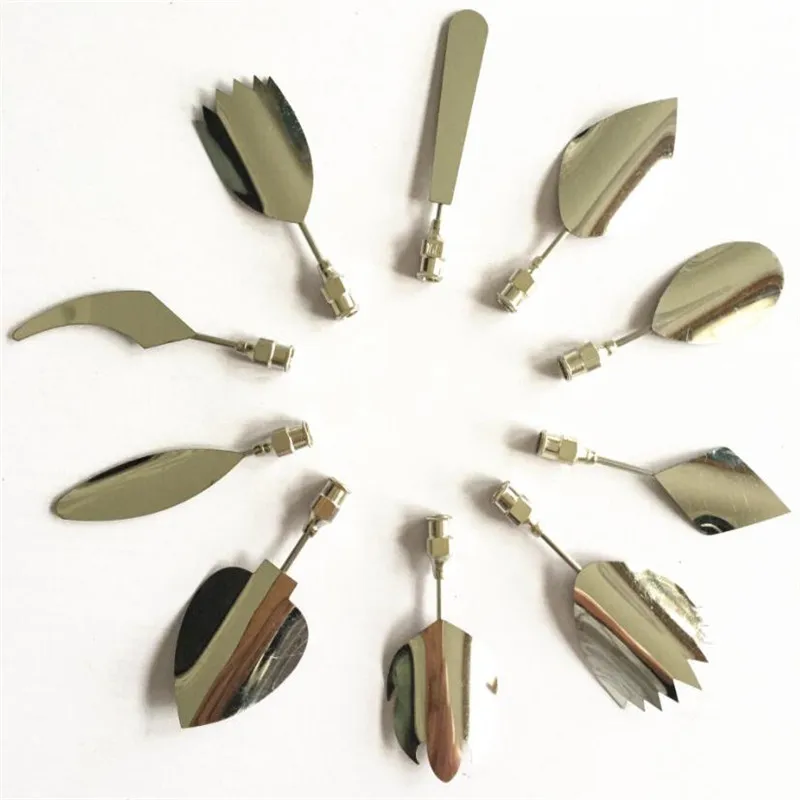This color photograph captures an array of various metallic objects meticulously arranged in a circular, clock-face pattern against a stark white background, devoid of any texture. The gleaming, silver objects are highly reflective, clearly mirroring their surroundings. Each object features a small socket-like base, suggesting they could be screwed into or attached to another component. Starting at the top and moving clockwise, the objects include a long, knife-like blade, a curved blade, a circular tool, a diamond-shaped implement, a rounded object with a pointed tip, a multi-pointed item, a spade-shaped piece, a more curved and pointed spade shape, a leaf-shaped tool, a sickle-shaped implement, and finally, an object shaped almost like a tulip at the 11 o'clock position. These meticulously designed tools, varying in size and shape, appear to be suited for delicate tasks, possibly culinary in nature, such as decorating cakes or smoothing frosting, each uniquely purposed for different intricate designs. The shadows cast by the objects add depth to the otherwise plain background.